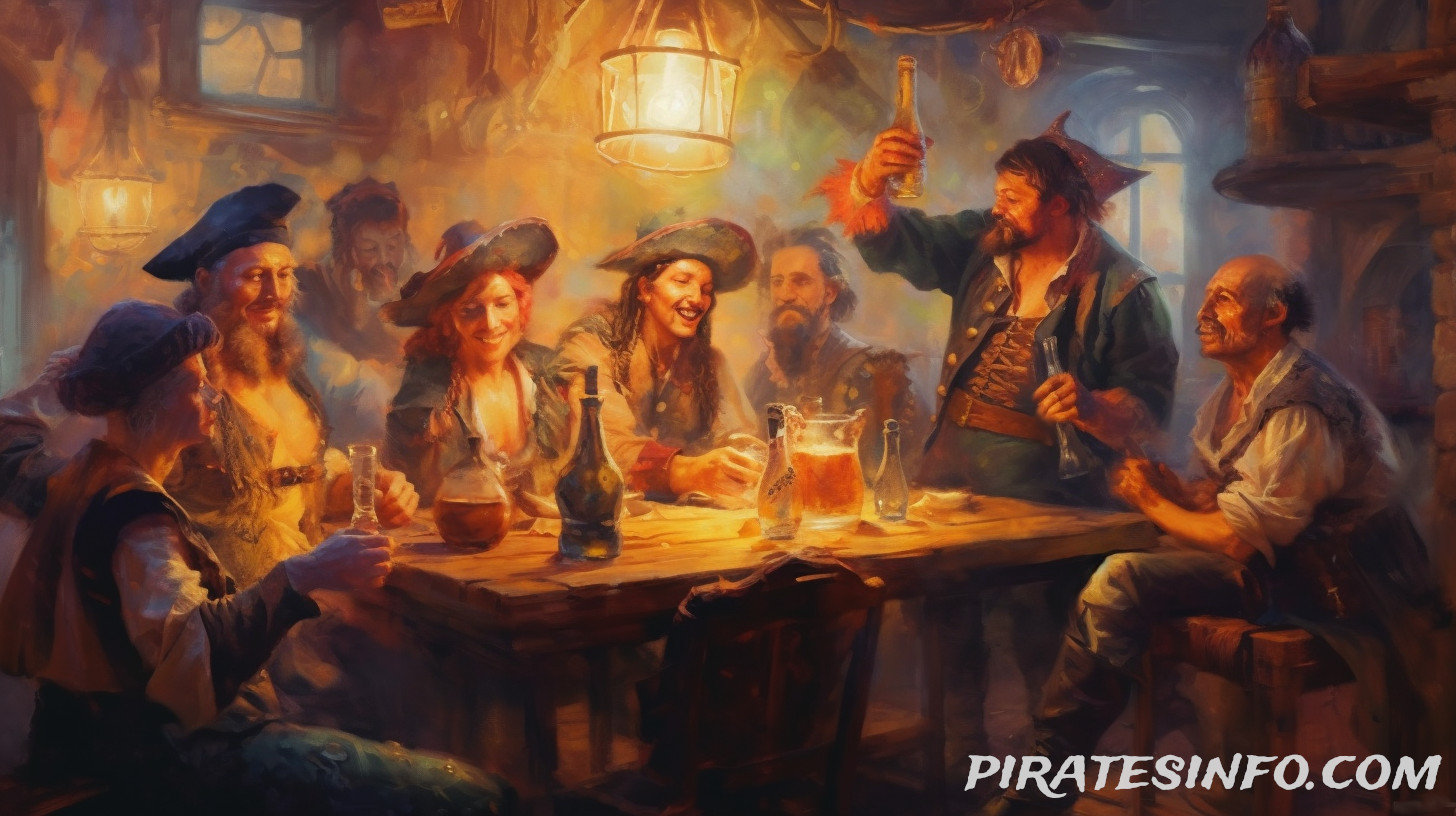The image depicts a lively indoor scene in what appears to be a tavern or pub, captured as a detailed painting or possibly a digitally created artwork. A wooden table, centrally located under a bright yellow hanging light, is surrounded by eight individuals, both men and women, who are dressed in pirate-themed attire, with the exception of a man on the right who wears no hat. The group, likely all Caucasian with light-tanned skin tones, are engaged in animated conversation, toasting and cheersing with various bottles and glasses of alcohol, including a noticeable pitcher of beer at the center of the table. One prominent figure, dressed in a blue outfit and standing, raises a beer in his right hand, adding to the sense of camaraderie and celebration. The bottom right-hand corner of the image features the text "PIRATESINFO.COM" in all capital letters and italicized, anchoring the lively scene and giving it a thematic label.